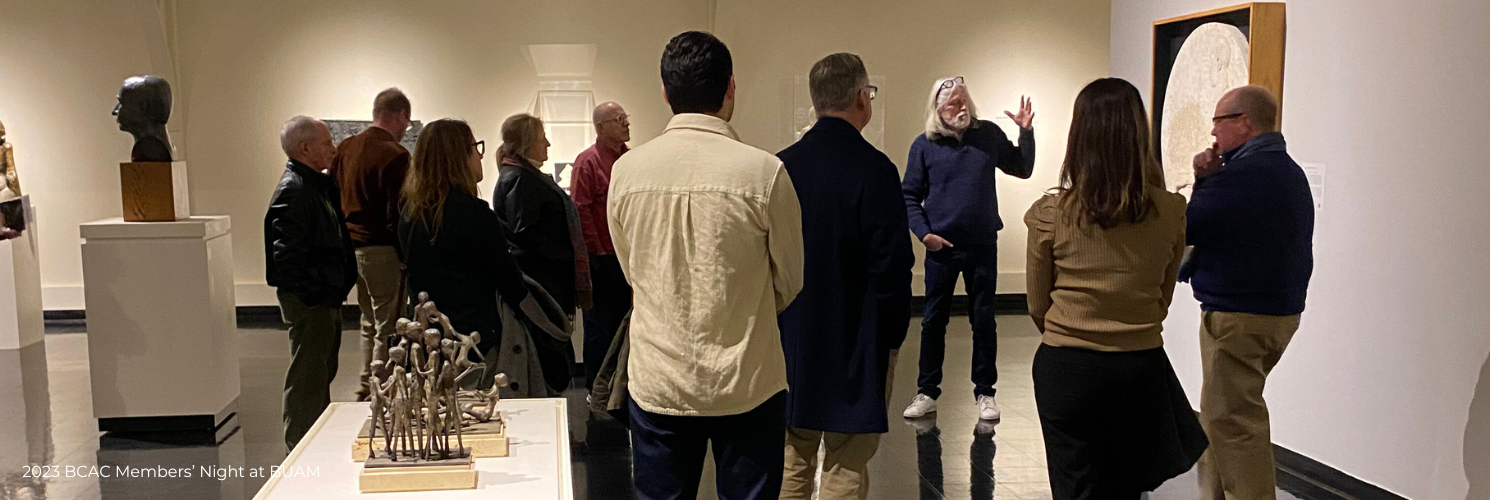The image depicts an art exhibition during Members Night at a museum, as stated by the text "2023 BCAC Members Night at Guam" located in the bottom-left corner. In the foreground stands an older man with white long hair, white facial hair, and glasses perched on top of his head. He is dressed in a blue long-sleeve shirt, jeans, and white sneakers. The man appears to be explaining or interpreting an art piece to a mixed group of men and women who have their backs to the camera. 

The focal point of the group’s attention is a framed object on the wall, which is not a typical painting but rather a disc-shaped piece, distinctly white in color. The man is gesturing towards this object with his left hand, further elaborating on its significance.

Surrounding this central scene are various other art pieces placed on pedestals. To the left, a bust faces away from the camera, obscuring its features. To the right, there are statues depicting a grouping of people, possibly warriors, lifting each other up, although the details are hard to make out. The setting is lively with the gathered crowd intent on the man’s explanation, encapsulating the engaged atmosphere of the museum event.